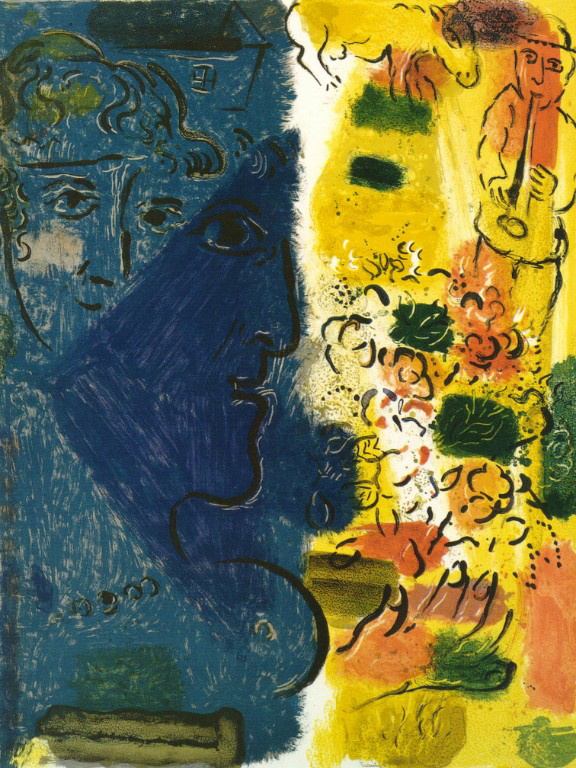This image features a modern abstract painting distinctly divided down the center, creating a contrasting dichotomy between the two halves. The left side predominantly showcases a melancholic blue theme, highlighted by two large faces. One face appears in a lighter blue hue, seen from the front with visible hair, while the other is darker blue, depicted in profile with only one eye, nose, mouth, and chin visible, and no hair. In the top left corner, there's a partial face of a woman, all contributing to the overall somber mood. The right side of the painting stands in vibrant opposition with a more cheerful palette of yellows, oranges, and greens, indicating a lively and upbeat atmosphere. This half features a poorly drawn human figure playing a trumpet, lending a festive feeling. Additionally, there's the lower half of an animal, possibly a cow or a horse, at the top right, symbolizing life and vitality. The bottom is adorned with greenish squiggles suggestive of bushes or flowers, further enhancing the lively and spirited essence of the right half.